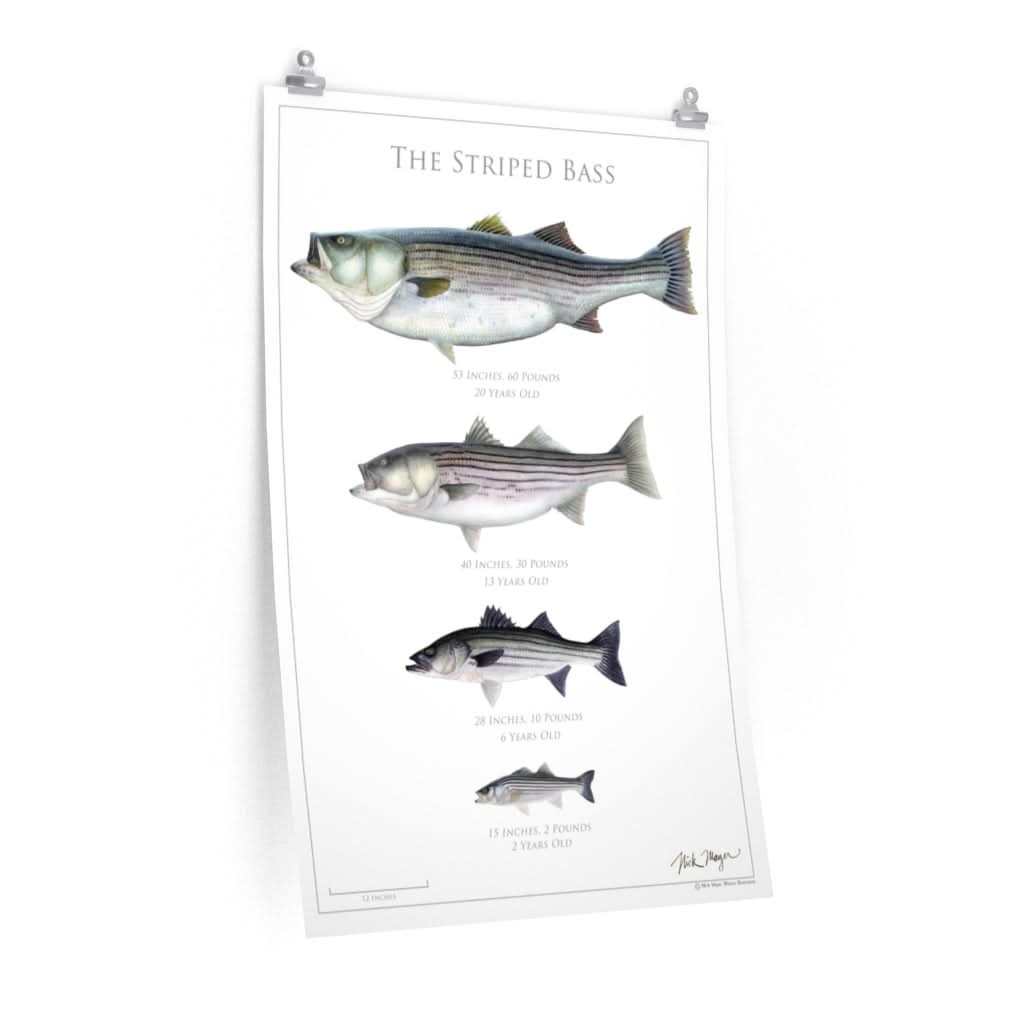This vertical poster, titled "The Striped Bass," showcases an infographic illustration of striped bass fish in a monochromatic color scheme with shades of grey, green, and black. The poster is held up by two silver clips at the top and framed by a thin black border. At the top, the title "The Striped Bass" is written in thin, serif font. The poster features four fish, arranged from largest at the top to smallest at the bottom, each with specific measurements and ages:

- The largest fish at the top measures 53 inches, weighs 60 pounds, and is 20 years old.
- Below it, the second largest fish measures 40 inches, weighs 30 pounds, and is 13 years old.
- The third fish down measures 28 inches, weighs 10 pounds, and is 6 years old.
- The smallest fish at the bottom measures 15 inches, weighs 2 pounds, and is 2 years old.

Each fish illustration is detailed, displaying subtle differences in size and coloration, with the largest fish depicted as more animated with its mouth slightly open. Additional design elements include a scale on the lower left corner to represent real-life proportions and the artist's cursive signature in the bottom right corner. The poster has a clean white background and appears to be a high-quality print, potentially meant for educational or decorative purposes.